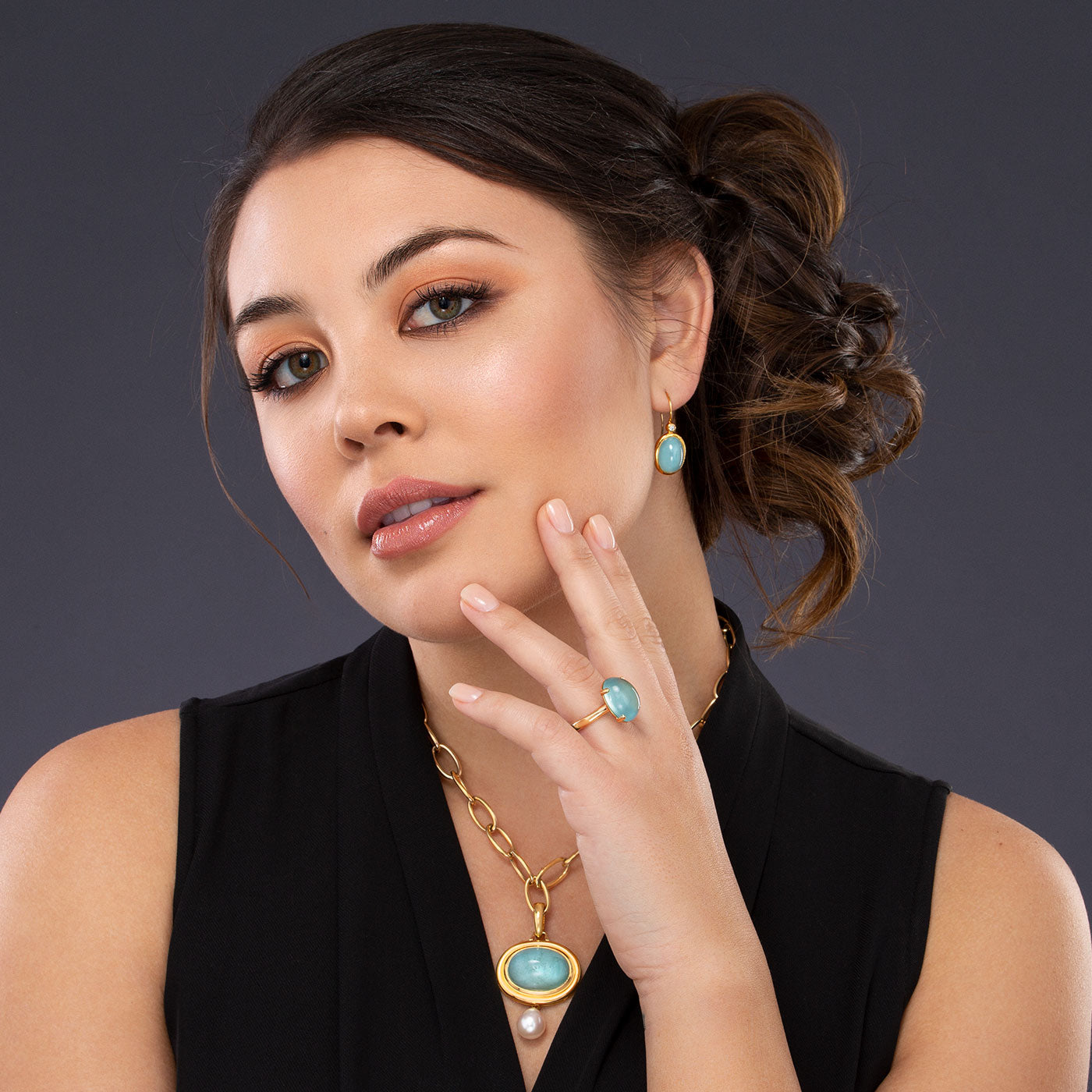The image features a striking portrait of a Caucasian woman set against a dark grey background. Her brown hair is elegantly styled, pulled up with numerous curls at the back, leaving a single tendril hanging down the right side of her face. Her makeup includes peach-colored eyeshadow and black eyeliner, which accentuate her brown eyes, and she wears light pink lipstick.

She is dressed in a black sleeveless garment with a deep V-neck. Her left arm is bent upward, with two or three fingers resting thoughtfully on her chin. She showcases a matched set of jewelry comprising an aquamarine gemstone encircled by gold. Her left hand displays an aquamarine ring with a gold band, while a similar oval aquamarine pendant, adorned with a pearl beneath and set on a gold chain, lies around her neck. An aquamarine earring with a gold latch adorns her left ear; her right ear is not visible in the image.

Overall, the focus is on the woman's sophisticated appearance and the harmonious arrangement of her light blue aquamarine jewelry.